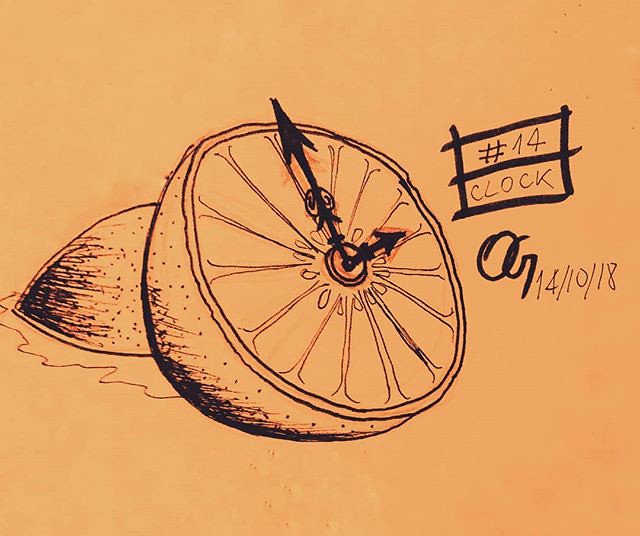This is a detailed pen and ink illustration on orange paper, with a few dark speckles in the background. The main focus is a sliced citrus fruit, resembling a grapefruit or cantaloupe, prominently displayed in the center. The fruit is realistically depicted, showing its wedges and dotted texture, and it has been cleverly transformed into a clock. Black clock hands, one pointing at 3 o'clock and the other at 12, are marked on the face of the fruit. Below the fruit, a puddle of juice is visible, adding to the realism.

To the upper right side of the image, there is a small square divided in half, featuring the pound symbol (#), with the handwritten text "number 14, CLOCK" beneath it. Additionally, there are several initials that appear to be "OG," along with the date "10/14/18." The other half of the citrus fruit is faintly visible behind the main one, contributing to the depth of the artwork. This unique piece is not only an artwork but also a creative representation of time through the medium of fruit.